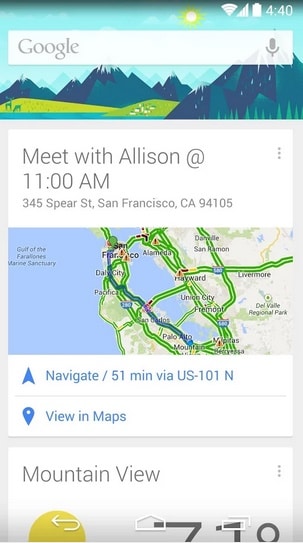The image on a phone screen depicts an animated Google search page with artistic drawings in the background. At the top, there are illustrated mountains and grassy areas, with deer drinking from a water source. The sun is shining brightly from the top, casting a golden hue over the scene. The sky is a teal color, with a few white clouds scattered across it. In the middle of the screen, "Google" is prominently displayed with a microphone icon in a search rectangle, indicating voice search capability.

Beneath the search bar, there is a reminder notification that reads, "Meet with Allison at 11:00 AM, 345 Speer Street, San Francisco, California, 94105." A map is visible below this reminder, showcasing the San Francisco area. The map highlights roadways in green, while one of the main roadways is depicted in a darker bluish-gray. Waterways are colored blue, adding contrast to the map. At the bottom of the screen, options for navigating and viewing directions in maps are readily available, marked by buttons labeled "Navigate," "Directions," and "View in Maps."